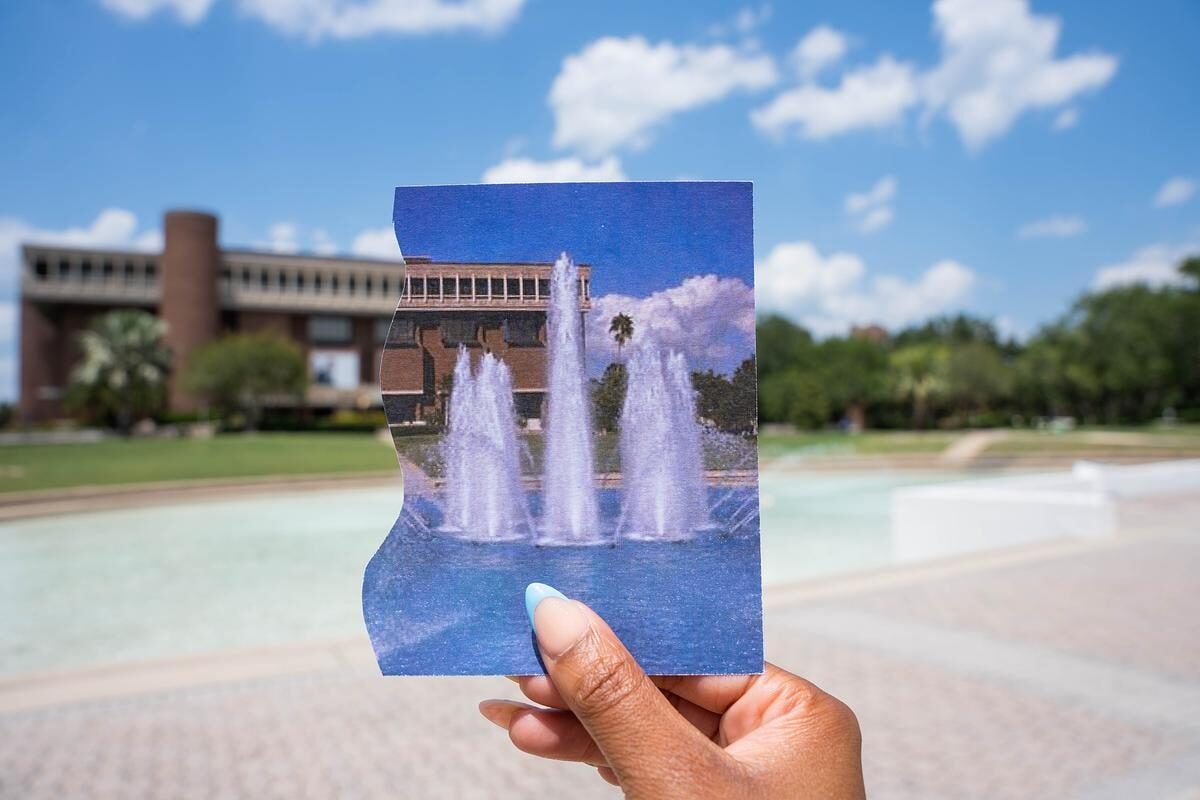A woman with long fingernails and somewhat dark skin holds up a photograph with her right hand, thumb and finger clasping a smoothly cut, curved edge. The photo depicts a pool with several fountains and a brown, possibly office building with many windows in the background. The main fountain spouts about six feet high, flanked by three shorter fountains on each side. She aligns the photo perfectly with the actual scene behind her, making it appear whole by covering the real fountains and the right side of the building. The sky above is a clear blue dotted with white clouds, echoed in both the photograph and the real background. Surrounding the structure, lush green trees complete the picturesque setting. In the foreground of the image, grayish-purple tiling leads to the pool’s edge.